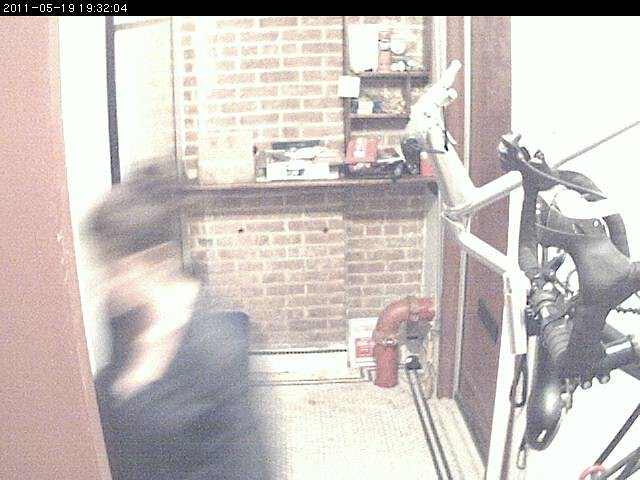This intriguing photograph, likely captured by a security camera, depicts a doorway scene marked with a timestamp in the upper-left corner. The timestamp reads "2011-05-19 19:32:04" in white text against a black border. The backdrop features a brick wall with white mortar lines, contributing to a rustic aesthetic.

In the foreground, a brown wooden door with a black mail slot occupies the right side of the image. Adjacent to the door stands a wooden shelf cluttered with various indistinguishable items. Additional smaller wooden shelves can be seen on the right-hand side of the image.

A bike rack is also visible, with a bicycle hanging from it, suggesting that this might be a transitional or storage area. Adding a dynamic element to the scene, a woman in a black low-cut top, her hair tied up in a bun, walks away from the doorway. Her movement introduces a motion blur, obscuring finer details of her appearance. The overall composition provides a narrative of a functional yet lived-in space, capturing a fleeting moment in time.